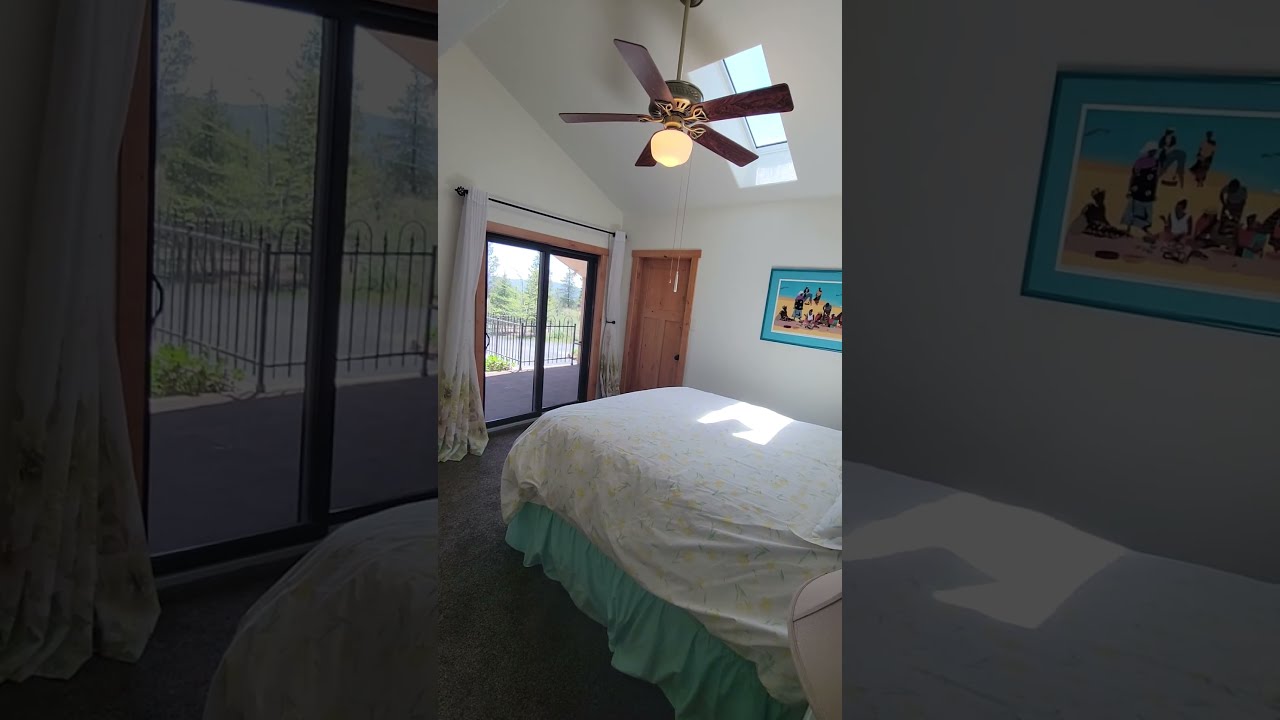The image depicts an intricately designed bedroom, creatively layered with a unique visual effect. At its core, there's a clearer, vertically centered photo of the room, laid over a blurrier version of the same scene in the background, creating a captivating splice effect down the middle. The bedroom features an elegant arched ceiling with a skylight that illuminates the space from above. Hanging from the ceiling is a brown wooden ceiling fan with five blades and a yellowish light bulb.

The focal point of the room is a full-size bed positioned toward the bottom corner. The bed is dressed with white sheets atop a turquoise bed skirt and a light bed cover adorned with a subtle yellow flower pattern. Adjacent to the bed, on one side, is a set of black-framed glass balcony doors with slightly drooping white curtains drawn to the side, revealing an outdoor balcony. Beyond the balcony, the view extends to a serene setting with trees and a water feature, possibly a lake.

On the wall behind the bed, there's a brown door with a small window near its top right corner, framed by white walls. To the right of the door hangs a framed photograph of several figures, bordered with teal matting that complements the scenic teal of the photo's sky. The room is suffused with natural light, creating a harmonious blend of indoor comfort and outdoor beauty.